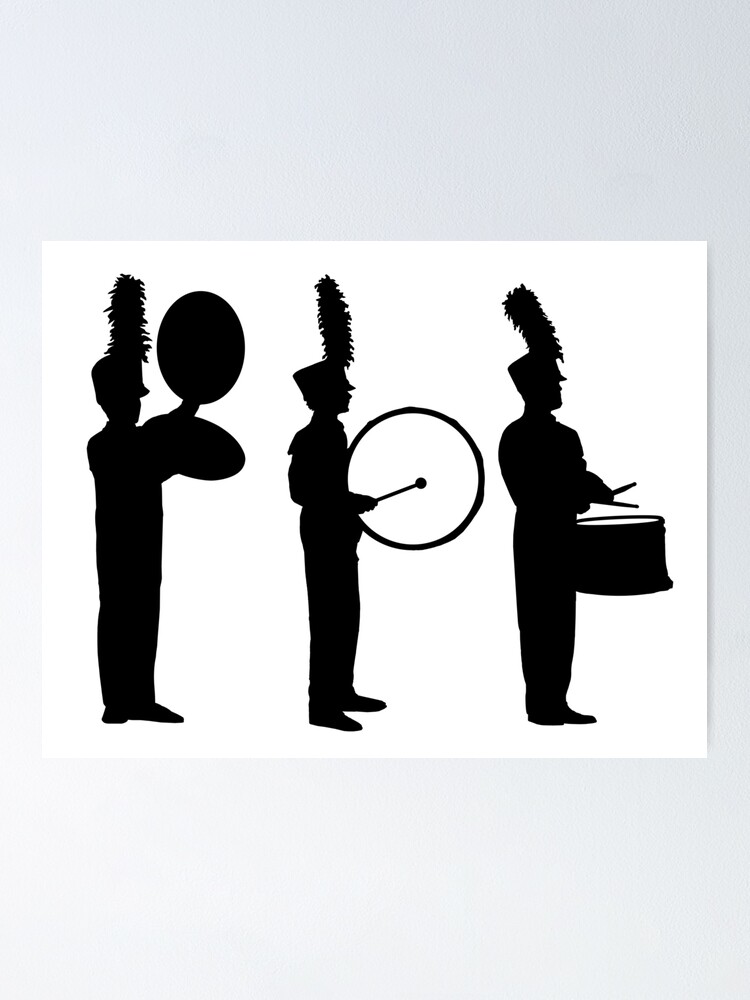The photograph shows the black silhouettes of three marching band members set against a large rectangular gray background, which acts as a banner or border, resembling a wall. The central image, also rectangular, has slightly longer top and bottom sides compared to the left and right sides. All three band members face the right, with the front member drumming on a small snare drum hanging from his hip. The middle member has a large bass drum positioned in front of his upper body, while the member at the back holds two cymbals. Each figure wears a traditional marching band hat adorned with feather plumes, though specific uniform details are indistinguishable. This gray background frames the silhouetted figures, emphasizing their stark, detailed outlines.